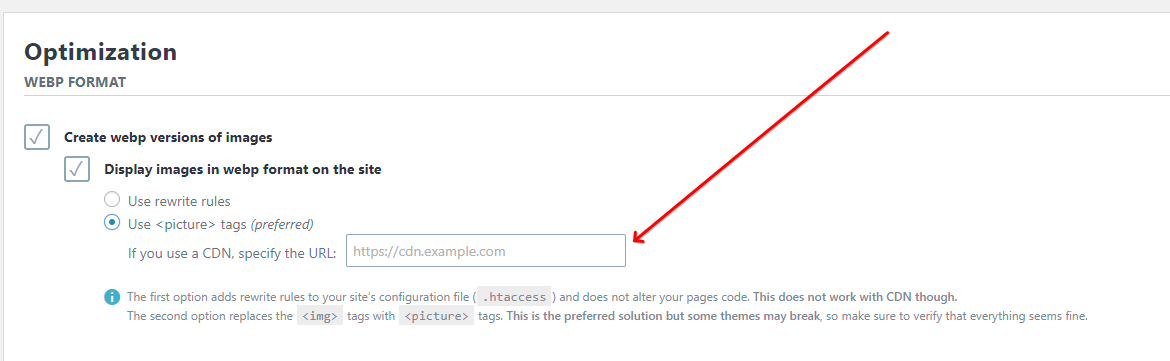This image is in landscape mode, and it appears to be a screenshot of a web optimization settings interface. 

### Detailed Description:
1. **Background**:
   - The top section of the image features a diagonal dark white stripe stretching from the upper left to the upper right corner and from upper left down to the lower left of the screen.

2. **Card Information**:
   - In the upper left corner of the card, the word "Optimization" is prominently displayed in bold black text.
   - Below "Optimization," the text "WEBP FORMAT" is written in capital letters with a light gray line underneath it.

3. **Checkboxes and Radio Buttons**:
   - There are two checkboxes:
     - The first checkbox is marked off, indicating it’s active. It is labeled "Create WEBP versions of images."
     - An indented subsection with another checked box reads: "Display images in WEBP format on the site."
   - Below these checkboxes are two radio buttons to choose from:
     - The first option says "Use rewrite rules," and the second option says "Use <picture> tags (preferred)." The second option with the <picture> tags has a filled green circle, indicating it’s selected.

4. **CDN Information**:
   - Further down, there's text that mentions, "If you use a CDN, specify the URL." Adjacent to this message is a green input box where a URL can be entered.
   - A large downward-facing red arrow points towards the input box, emphasizing where to type in the URL.

5. **Explanatory Note**:
   - At the bottom, there is an icon resembling an eye, followed by a note stating: "The first option adds rewrite rules to your site's configuration."

This structured and comprehensive caption outlines the key elements of the image in detail, providing a thorough understanding of the interface depicted.